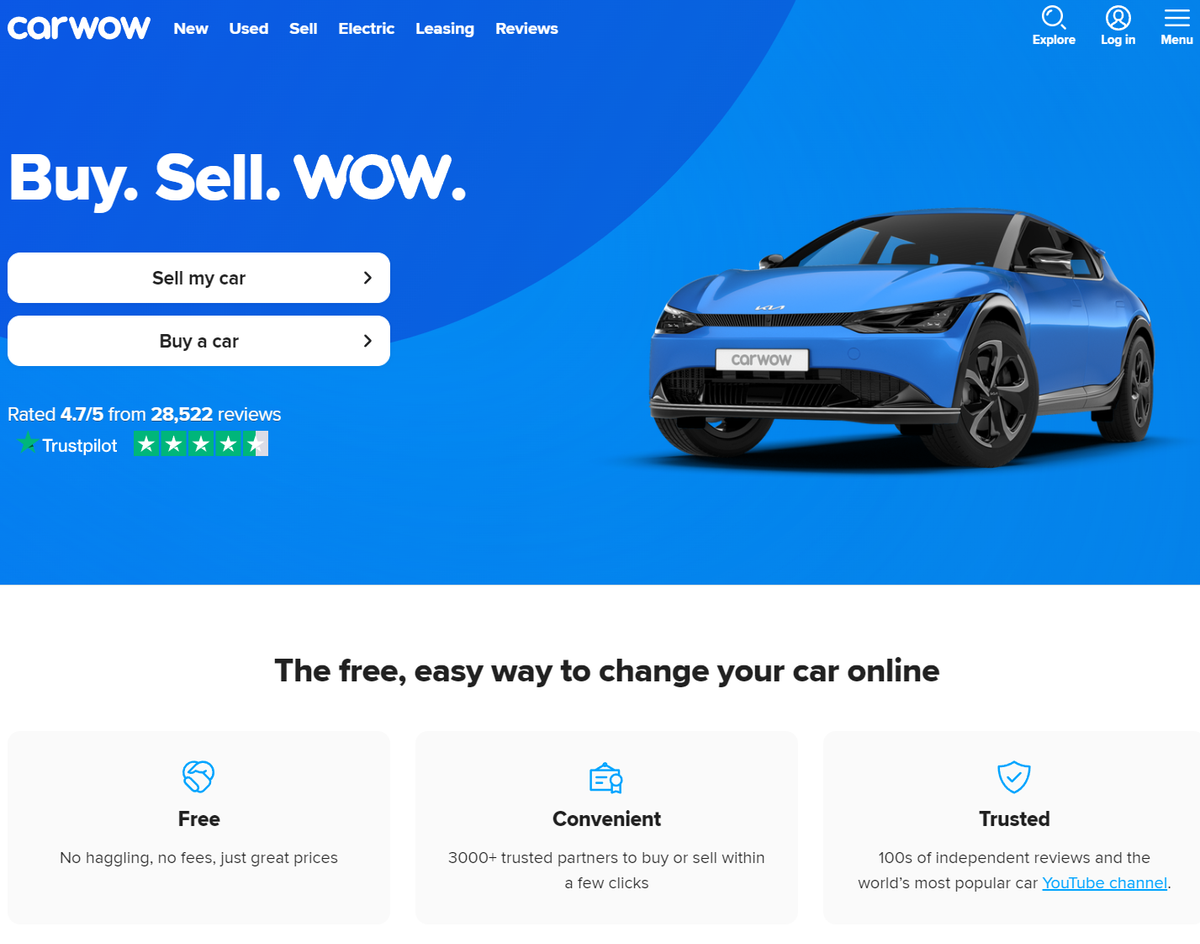The image depicts a webpage header styled with a blue rectangular banner, prominently displaying "CarWow" in white letters, along with several menu options: "New," "Used," "Sell," "Electric," "Leasing," "Reviews," "Explore," "Login," and "Menu," all stretching from the left to the right. Directly beneath this header, aligned to the left, the text reads "Buy. Sell. Wow." in sequence. Below this slogan, two white rectangular buttons with black text offer the options "Sell My Car" and "Buy a Car." 

Further down, the banner continues with a blue background, featuring the text "Rating 4.7/5 from 28,522 reviews" in white letters. This is followed by a green star icon and the word "Trustpilot" in white. Accompanying this are green squares each containing grey stars, visually representing a four and a half-star rating from Trustpilot.

To the right side of the banner, there is an image of a blue four-door car, bearing a "Car Wow" logo on its front license plate area. Beneath the banner and next to the car, the text reads "The free, easy way to change your car online." Additionally, from left to right at the bottom, the terms "Free," "Convenient," and "Trusting" are outlined, each supplemented with explanatory paragraphs in fine print.